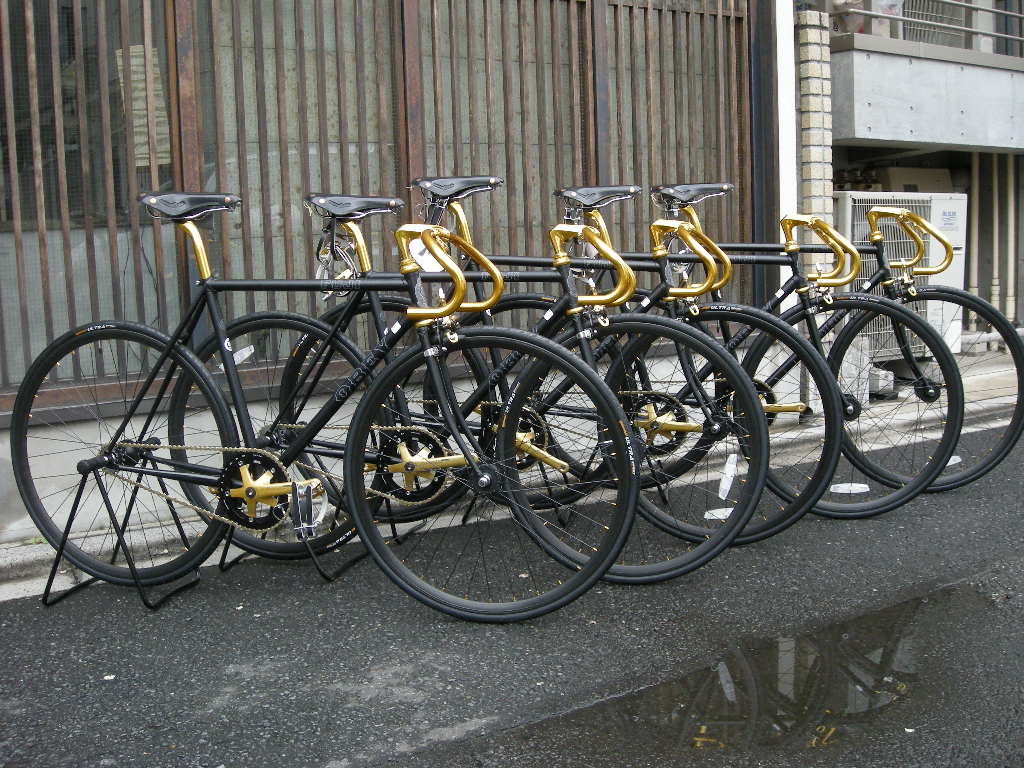This photograph features five identical racing bicycles, each with a sleek black metal frame and notable gold accents. The golden components include the handlebars, the seat posts, and the crankshafts for the pedals. These bicycles are securely mounted on portable kickstands designed to elevate the back wheels and keep them standing upright.

The setting appears to be an outdoor, industrial-style area. In the background, there is a building with metallic bars and girders, as well as a visible air conditioning unit. The scene includes a sidewalk and a street, which has visible puddles, suggesting it has rained recently. This water accumulation has created a large mud puddle on the road. The bicycles are parked neatly in a row along the curb, likely in a designated bike stand area. The overall composition suggests a neatly ordered yet gritty urban environment.